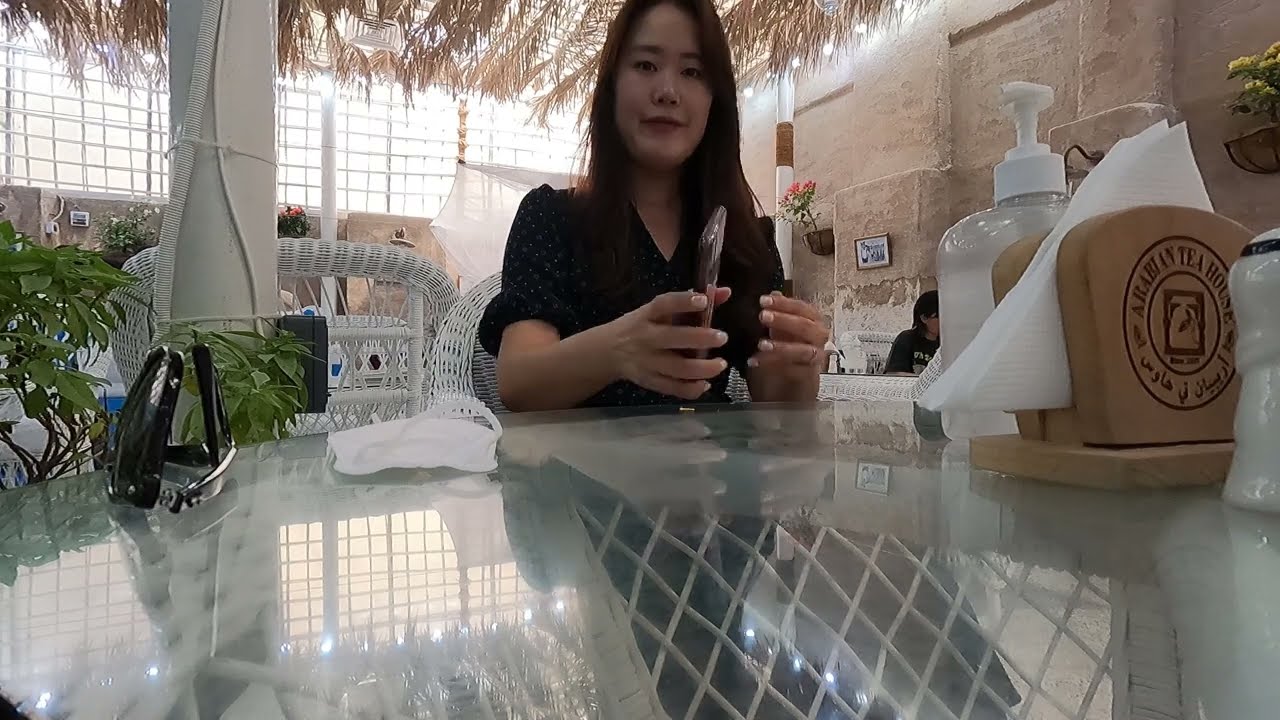The image captures a young Asian woman, possibly in her late 20s, seated at the center of a glass table. She is wearing a black dress adorned with white polka dots and short sleeves, and is holding a tan-colored, flat smartphone in her right hand. Her gaze is directed towards the camera, which appears to be positioned on the table in front of her. In the background, a bright and airy environment is discernible, with a straw roof overhead and several white wicker chairs and additional tables occupied by other people. The setting is further characterized by a beige and white wall, illuminated brightly, and a large window occupying two-thirds of the background with some blue signage above an obscured figure. To her right, a green potted plant sits adjacent to a white pillar extending to the ceiling. On the table, among other items, are a hand lotion bottle, a wooden napkin holder branded with the words "Arabian Tea House," a pair of sunglasses, some tissues, and a black device, likely a camera. The overall scene suggests a tranquil café or tea house, highlighted by meticulously detailed décor and ambient lighting.